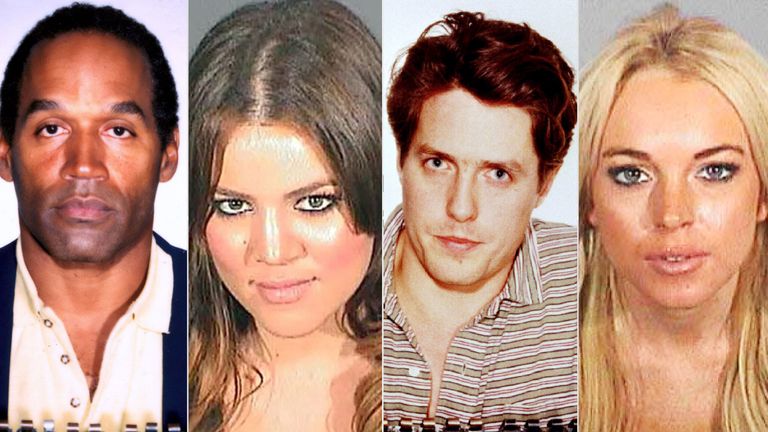This image is a composite of four mugshots featuring notable Hollywood figures, each presented in color and formatted as individual panels placed side by side. From left to right, the first photograph is of O.J. Simpson, recognizable for his dark hair and serious expression. Next is a brunette woman with a clear complexion, possibly Khloe Kardashian, though the identity is uncertain. The third image is a mugshot of Hugh Grant, identifiable by his light skin and reddish-brown hair; he is wearing a collared, vertically striped shirt. Lastly, the fourth panel showcases Lindsay Lohan, who appears with blonde hair and a similarly serious demeanor. Each image exhibits the subject facing forward against a plain background, with both men reportedly holding items featuring noticeable black ridges. Despite the differences in appearance and attire, the images share a consistent format, emphasizing a uniform layout and solemn mood reflective of their context.